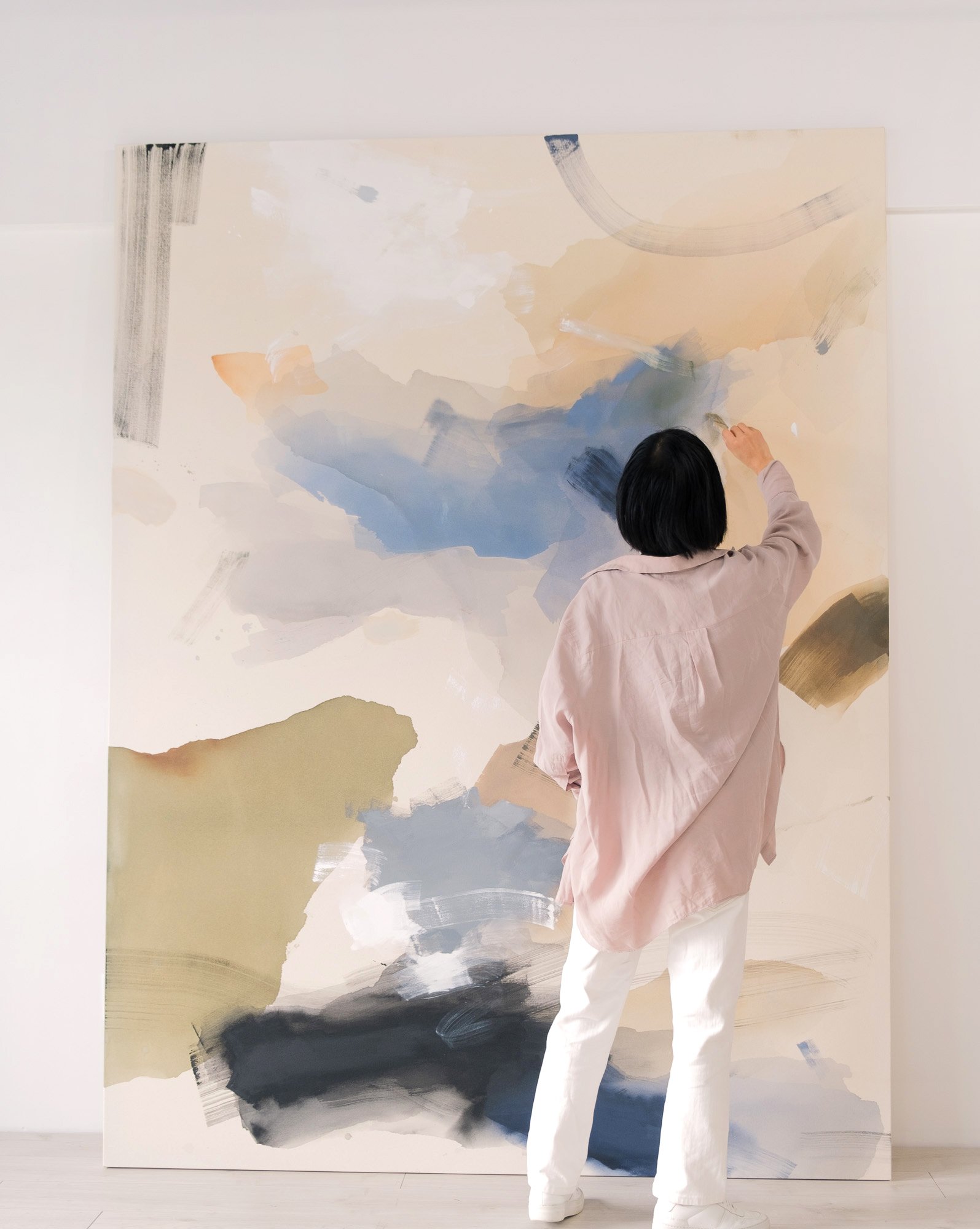In this captivating photograph, a young woman, who appears to be around five foot one with black hair, is deeply engrossed in painting a large, abstract canvas that is about three times her size. The canvas is propped up against a stark white wall, which is protected by a white paper or poster. The light gray wooden flooring beneath her adds a modern touch to the setting. Dressed in white pants, white shoes, and a long-sleeve pink (or mauve) button-up shirt that's open, the artist stands with her back to the camera, her arm raised as she delicately applies blue paint with a light brown paintbrush. The canvas itself is a vibrant medley of different colors and shapes, lacking any definitive form but featuring various blobs and swirls of tans, dark blues, light blues, whites, oranges, and black, including a prominent black spot at the bottom and a blue spot directly in front of her. The scene exudes creativity and focus, hinting at the beautiful, abstract masterpiece in the making.